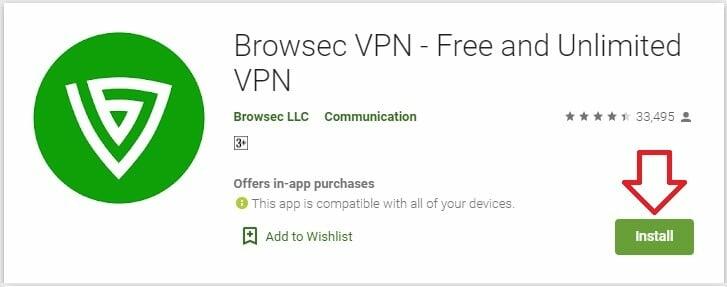A promotional banner for BrowseSecVPN is displayed, resembling the size of a typical online advertisement. The left portion of the banner prominently features a logo: a green circle encompassing a downward-facing white triangle with a maze-like design inside it. Adjacent to the logo, text reads "BrowseSecVPN - Free and Unlimited VPN," followed by the publisher’s name, "BrowseSec LLC Communication." 

Moving to the right side of the banner, a star rating system is shown, with four fully colored stars and one half-colored, accompanied by the number "33,495" indicating user reviews. Below this, an icon of a person is visible.

Further down on the right, there's a '3+' box denoting compatibility, alongside text stating "Offers in-app purchases." Another green circle—signifying that the app is "compatible with all of your devices"—is displayed, followed by a ribbon icon with a plus symbol that indicates the option to "Add to Wishlist."

Located at the bottom right corner is a green "Install" button with white text, highlighted by a digitally added arrow pointing towards it, encouraging installation.